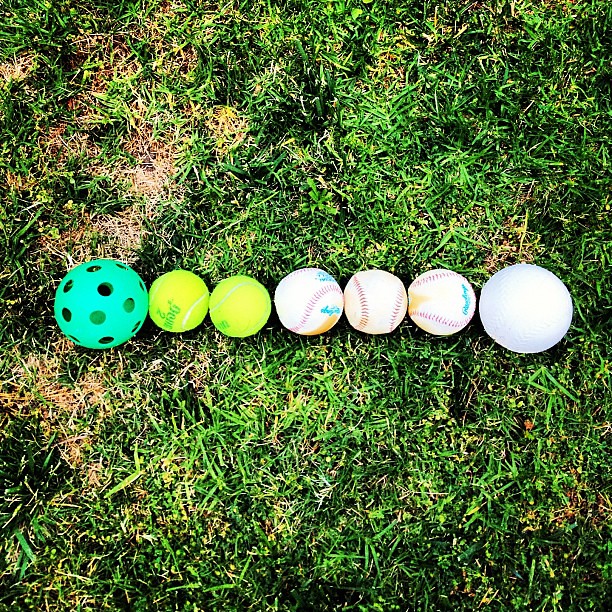The image displays a square plot of grass that serves as the background, with sections of both lush green and patches of gray or brown, dying grass scattered throughout. Horizontally aligned from left to right in a straight line, there are seven sports balls, each touching the next. Starting on the far left, there is a greenish-teal wiffle ball characterized by its holes. To the right of it, there are two tennis balls of a typical bright yellow hue, marked with a green logo. Following these are three baseballs, each featuring red stitching and a combination of blue and gray logos, although one of the baseballs has its logo obscured. On the far right is a larger white ball resembling a softball, notably absent of any stitching or logos. Together, these balls rest on the variously colored grass, creating a visually detailed and descriptive scene.